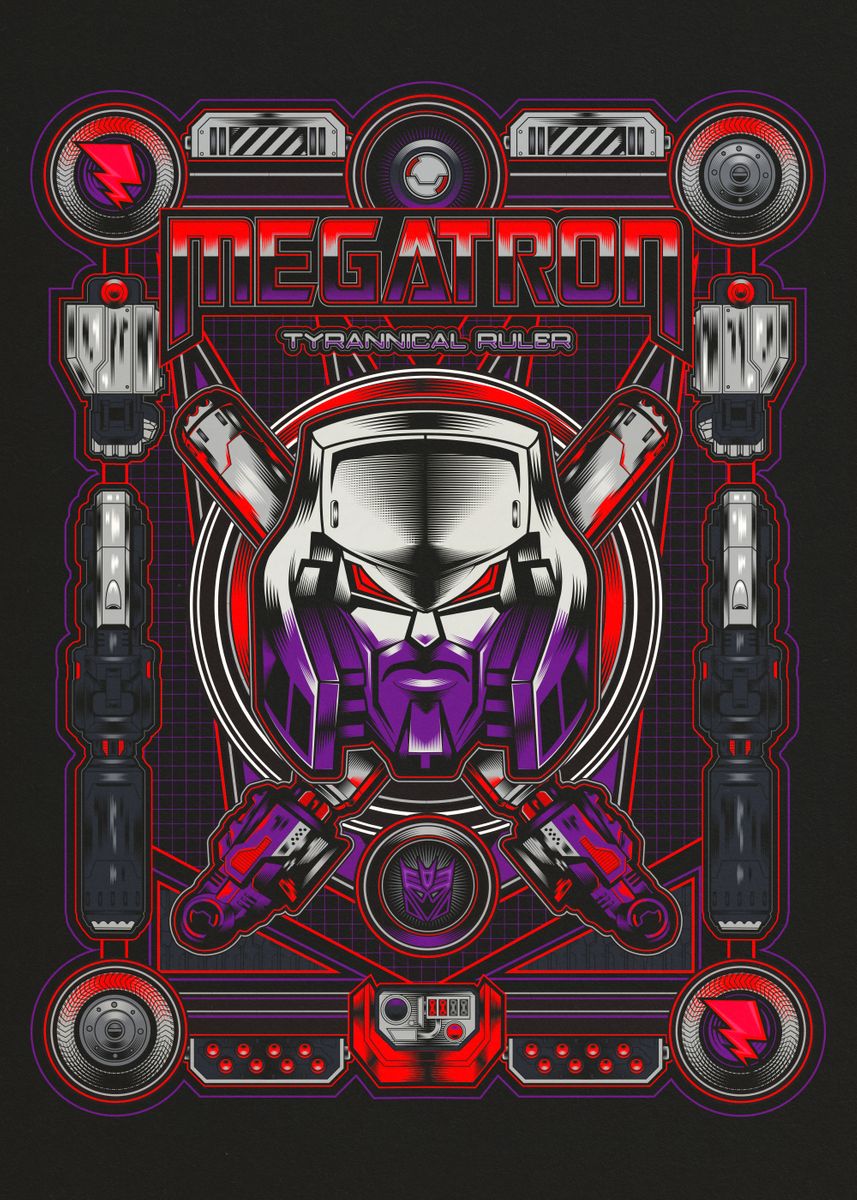This poster features a striking, cartoon-style image of Megatron from Transformers. At the top, bold multicolored letters transitioning from red to purple spell out "Megatron," with the subtitle "Tyrannical Ruler" in smaller purple letters below. Dominating the center is a fierce depiction of Megatron's face, its colors shifting between silver metallic gray and purple. The face glares directly at the viewer with red, squinting eyes. Surrounding Megatron's head is a rectangular frame formed from various robot and car parts, including wheels, lightning bolts, speed dials, knobs, robotic fists, and battery-like components, all in a mix of silver, black, red, and gray hues. Red circles accent some corners of the frame, heightening the dramatic effect. Additionally, metallic poles extend from behind Megatron's shoulders, completing the imposing and detailed mechanical aesthetic of the poster.